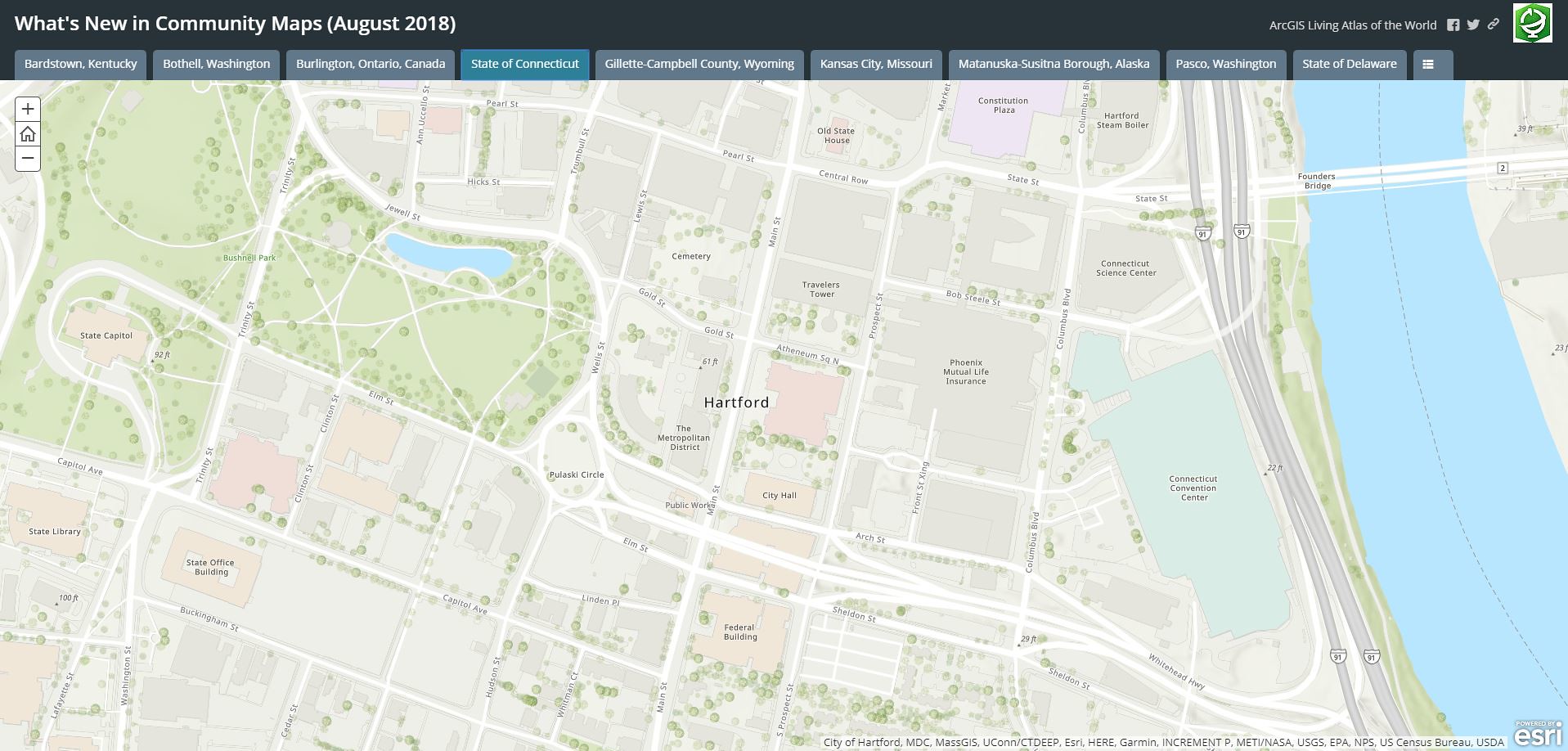A horizontally oriented, pastel-colored map illustrating a community, featuring a river along the right edge bordered by Interstates 31 and 51. A park is located in the top left corner. A house icon with zoom in and out buttons overlays the map, which is titled "What's New in Community Maps August 2018" in the browser bar. The active blue tab indicates the state of Connecticut. At the map's center is Hartford, the capital of Connecticut, with labeled streets, a convention center, and other significant landmarks. The top right corner displays a green and white logo. Various parts of the map include black text indicating their position and use.